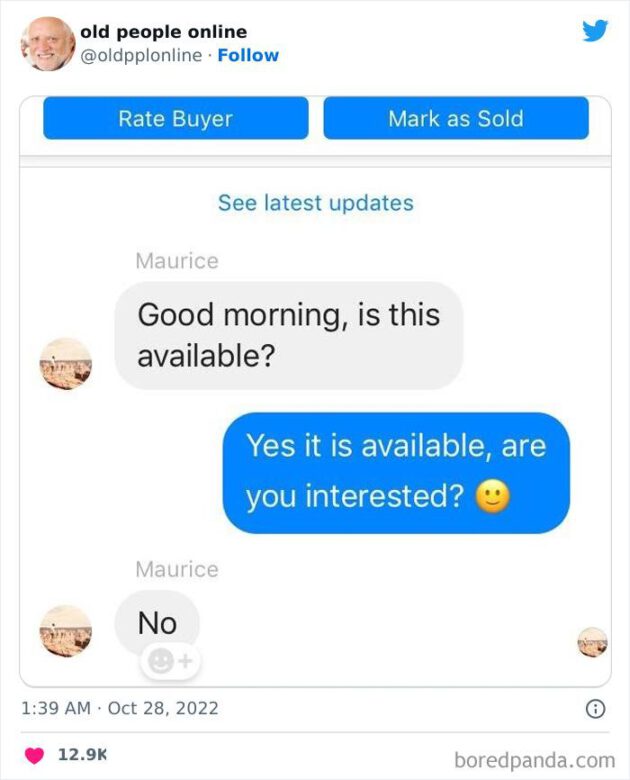The image showcases a screenshot from the website BoredPanda.com. At the top of the page, there is a small circular profile picture with the username "Old People Online." Directly beneath, there are blue buttons labeled "Rate Buyer" and "Mark as Sold." A Twitter icon is visible in the top right corner of the screen.

Below this header is a white dialogue panel displaying a series of messages between users. At the top of this panel is a clickable blue link that reads "See Latest Updates." 

The conversation begins with a user named Morris asking, "Good morning, is this available?" A response follows: "Yes, it is available. Are you interested? 😊" Morris then replies, "No." This exchange is timestamped at 1:39 AM on October 28, 2022, as indicated in the bottom left corner of the screen. Notably, this humorous interaction has garnered 12.9 thousand likes.